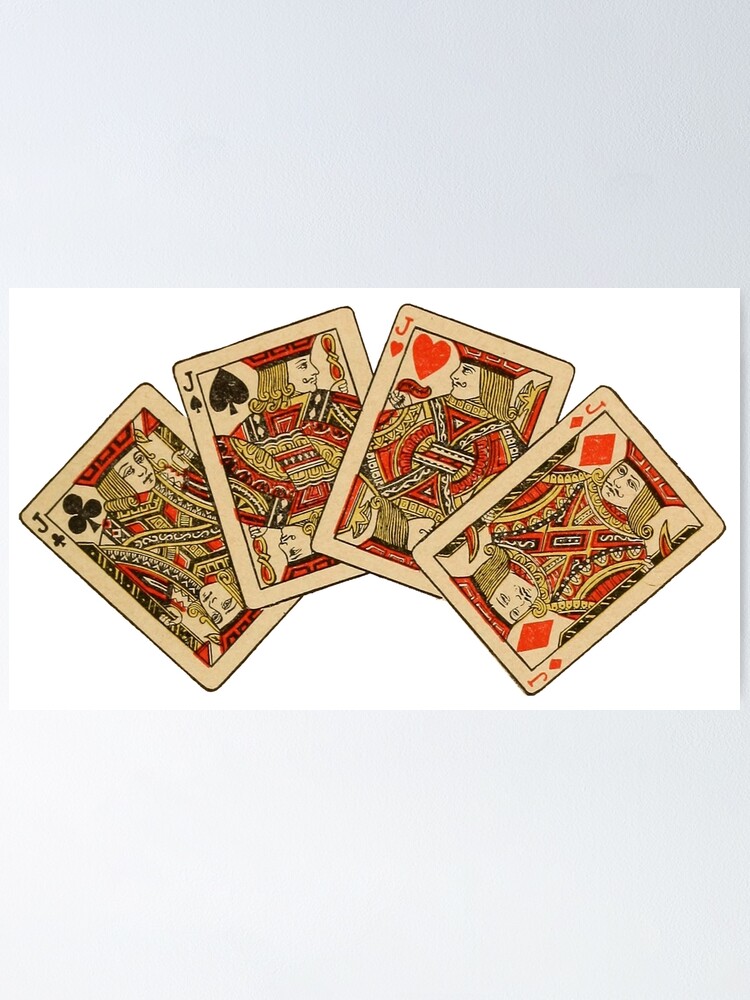This photo showcases a set of four playing cards, each featuring a different Jack: the Jack of Clubs, the Jack of Spades, the Jack of Hearts, and the Jack of Diamonds. The cards are arranged in a semi-circle on a plain white background, resembling how they might appear if held in a fanned-out hand. The cards appear aged, with a tan or beige hue indicating their older nature, and display designs in red, black, yellow, and white. Each Jack figure is distinct, some adorned with mustaches, and all wear red hats. The Jack of Clubs has long, curly yellow blonde hair. The Jacks of Clubs and Spades face to the right, while the Jacks of Hearts and Diamonds face to the left. The detailed artwork on these cards has a somewhat faded appearance, enhancing their vintage charm.